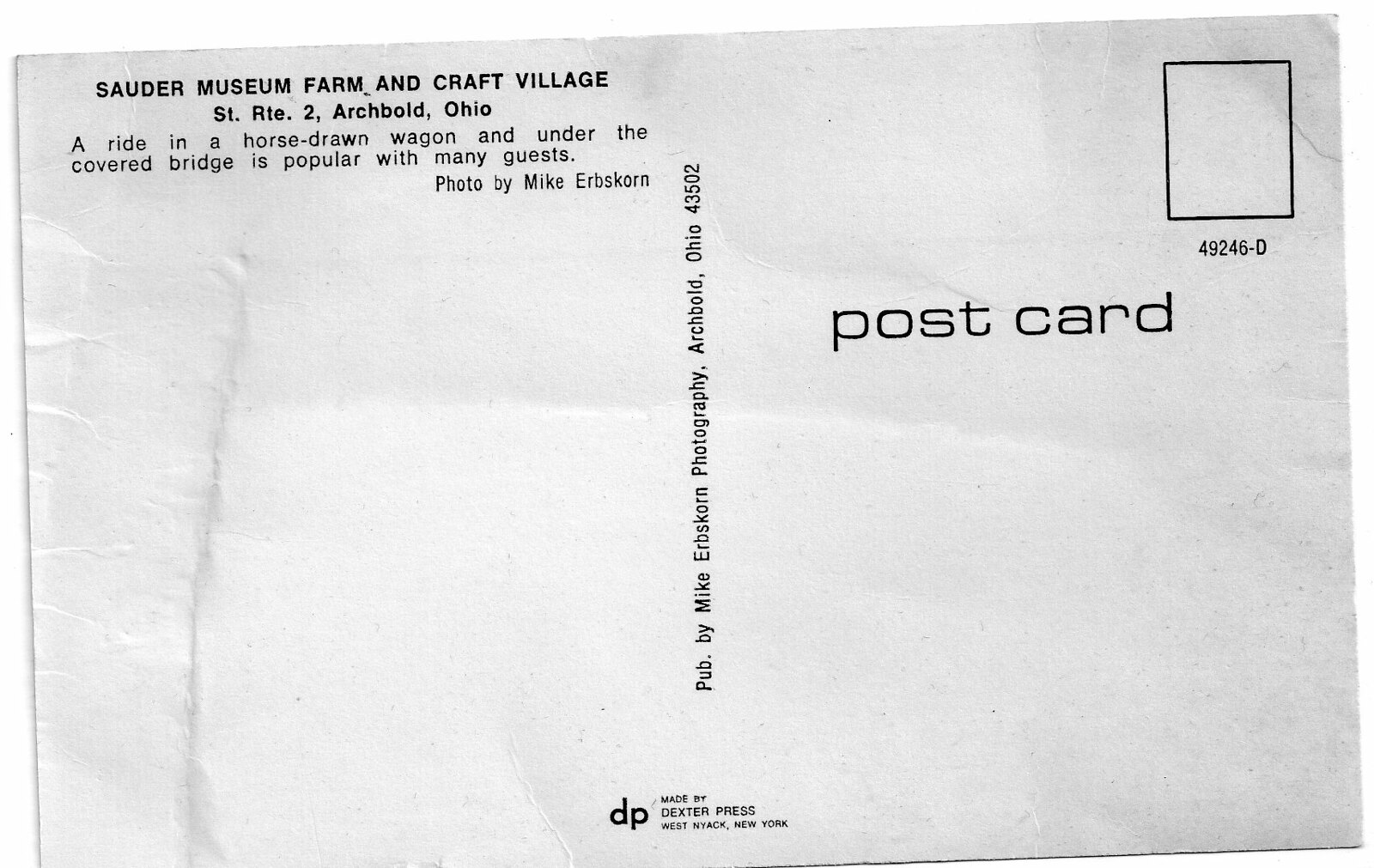This image shows the backside of a slightly tilted, worn, and dated black and white postcard. The postcard's back is white with black text. In the top left corner, "Souder Museum Farm and Craft Village, State Route 2, Archbold, Ohio" is prominently printed. Directly below that, there is a caption reading, "A ride in a horse-drawn wagon and under the covered bridge is popular with many guests." This photo credit, attributed to Mike Erbskorn, suggests he both took and published the photograph, as indicated by the vertical center-aligned text "Pub by Mike Erbskorn, Photography, Archbold, Ohio, 43502." On the right side, a designated rectangle marks the spot for a stamp, labeled with "49246-D" beneath it, followed by the word “Postcard.” At the very bottom center of the card, it reads "Made by Dexter Press, West Nyack, New York."